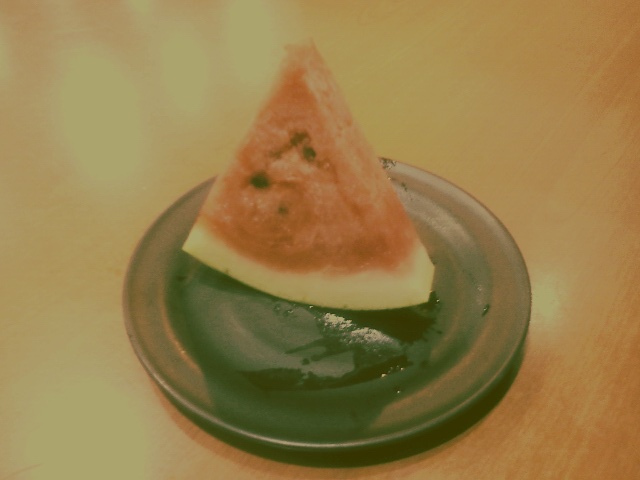This photograph showcases a triangular slice of watermelon set upright on its white rind on a round, brown ceramic plate. The vibrant red flesh of the watermelon is dotted with a few black seeds, and there's a hint of green where the rind meets the flesh. The plate features a distinctive black discoloration at its center. The setup rests on a brown wooden table with a yellowish tint.